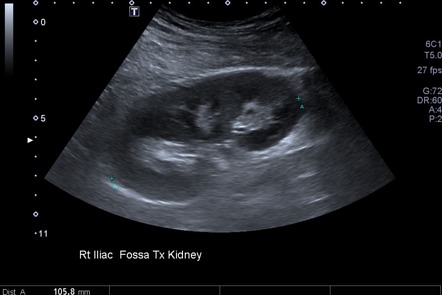This image is an ultrasound scan focusing on the right iliac fossa space, specifically targeting the kidney. The background of the image is predominantly black, highlighting the greyish ultrasound area with white streaks and notches. At the center of the image, there’s a notable grey oval shape indicating the kidney. Below this central section, the label reads "RT Iliac Fossa TX Kidney". 

On the left side of the image, there's a vertical scale numbering from 0 at the top and counting down to -11, with the middle number marked as 5. An arrow points to a spot just below the number 5, indicating a dot of interest in that area. 

On the right edge of the image, various trackable data points are visible: at the top, "6C" and "T5" are displayed, followed by "27FPS". Further down, though some text is cut off, discernible parts read "G; 72", "DR; 60", "A; 4", and "P2". In the bottom left corner, the number 105.8 is visible. 

This detailed depiction provides a comprehensive understanding of the ultrasound image, capturing all prominent details and annotative marks.